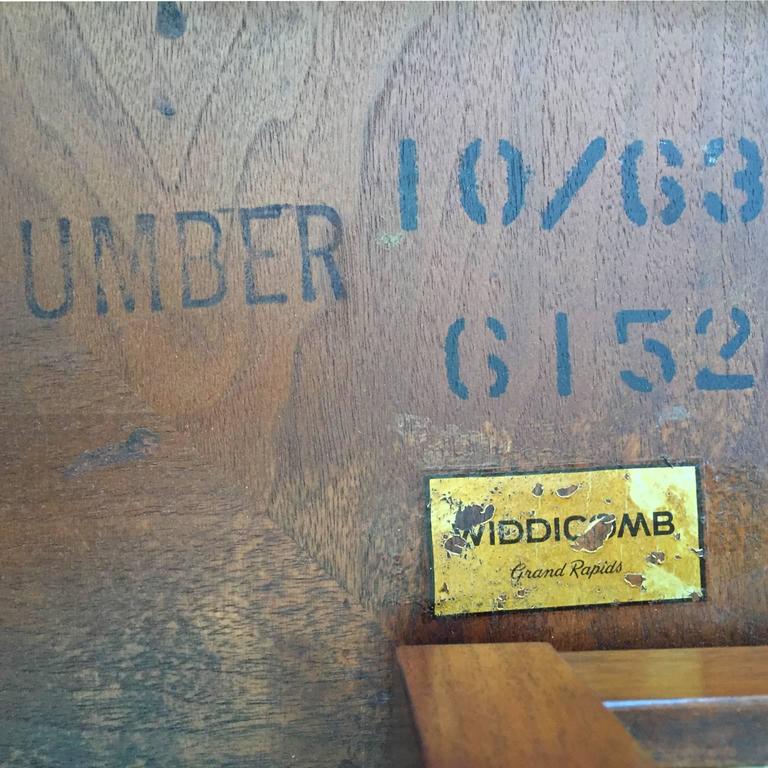The close-up image reveals what appears to be the underside of a medium brown, varnished wooden piece of furniture, likely a table or end table. The wood surface is aged and worn in places, featuring several stamps and a damaged gold plate with black text. The more legible elements of the stamps include the word "Umber," and numbers such as "10-63" and "6152," suggesting a manufacturing or tracking process. The gold plate, though worn, reads "Widdicombe Grand Rapids." The image also shows, from the angle, a table leg extending downward, reinforcing the likelihood that this is the underside of a table. The overall coloring of the image includes shades of brown for the wood, black for the text, and gold for the plate.